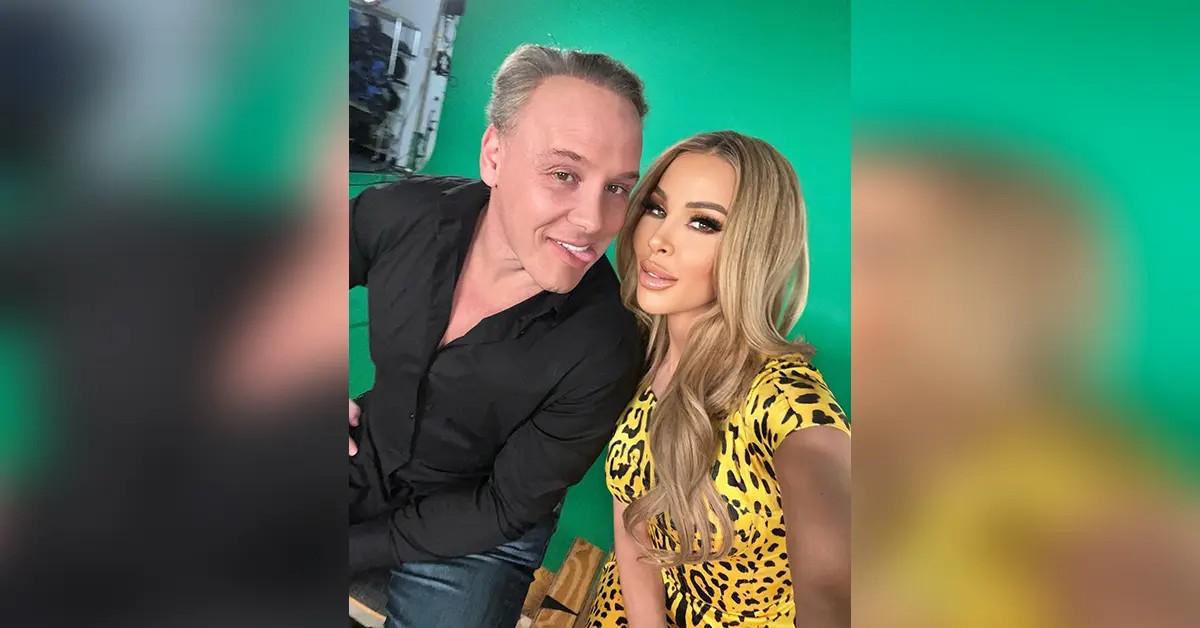This horizontally-oriented image is divided into three vertical sections, with the middle section slightly larger than the left and right. The central part features a man and a woman, possibly celebrities, standing against a green background that might be a green screen.

The man, positioned on the left, has short grayish hair and is wearing a black button-down shirt and dark-colored pants, likely blue jeans. His body is angled somewhat to the left, but his head is turned toward the woman next to him. He appears to be sticking his tongue out slightly and is leaning to the right. His right arm extends out of the image to the left just below the shoulder, while his left arm disappears off the frame at the wrist.

The woman, located on the right, is leaning slightly into the man. She has long, wavy blonde hair that cascades down the left side of her chest. She is wearing pink lipstick and a yellow top or dress with a black cheetah print. Her body extends out of the image below the waist, with both arms also exiting the frame at the bottom. Observers noted that she appears to have heavy makeup and possibly cosmetic enhancements like lip fillers and Botox.

The left and right parts of the image are blurred extensions of the main photograph. The left section contains a mix of black, green, and light colors, seemingly a distorted version of the man. The right section, with hues of yellow and green, appears to be a blurred replica of the woman's right side. This blurring effect might be a result of formatting the vertical shot to fit a horizontal space.